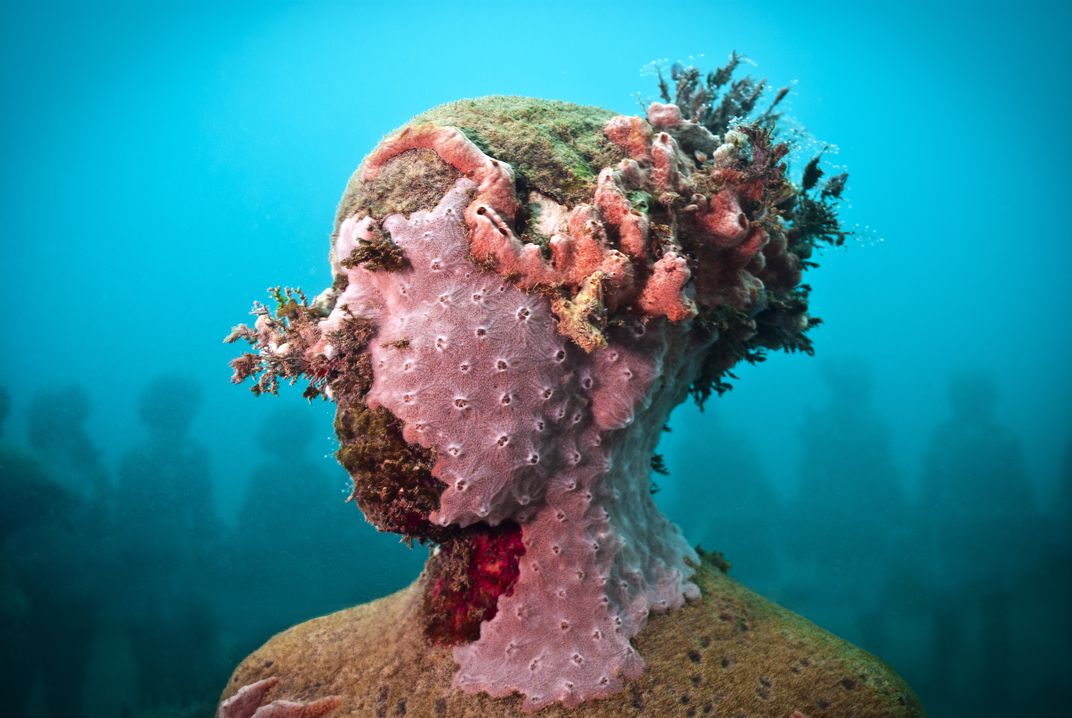In this surreal and vividly colorful image, we see the left side profile of a woman's head and shoulders, her features obscured by an elaborate, textured mask. The mask, in shades of pink, has numerous perforations and intricate brown outlines marking the eyes, nose, and mouth. Atop her head, where hair would typically be, is a whimsical, patterned cap with hair protruding from the back. This cap, alongside other plant-like elements, suggests an immersive underwater theme. The woman’s head and shoulders are enveloped in what appear to be sea plants, moss, and corals in a mix of greens, whites, pinks, and yellows, which give the image a highly texturized and organic feel. The background, a bright aqua blue, features blurred, shadowy figures that convey an impression of an underwater scene or a deep sea environment. The overall pastel palette of pinks, blues, and greens, combined with the three-dimensional realism of the textures, underscores the artistic and possibly CGI-rendered nature of this unique, imaginary portrait.